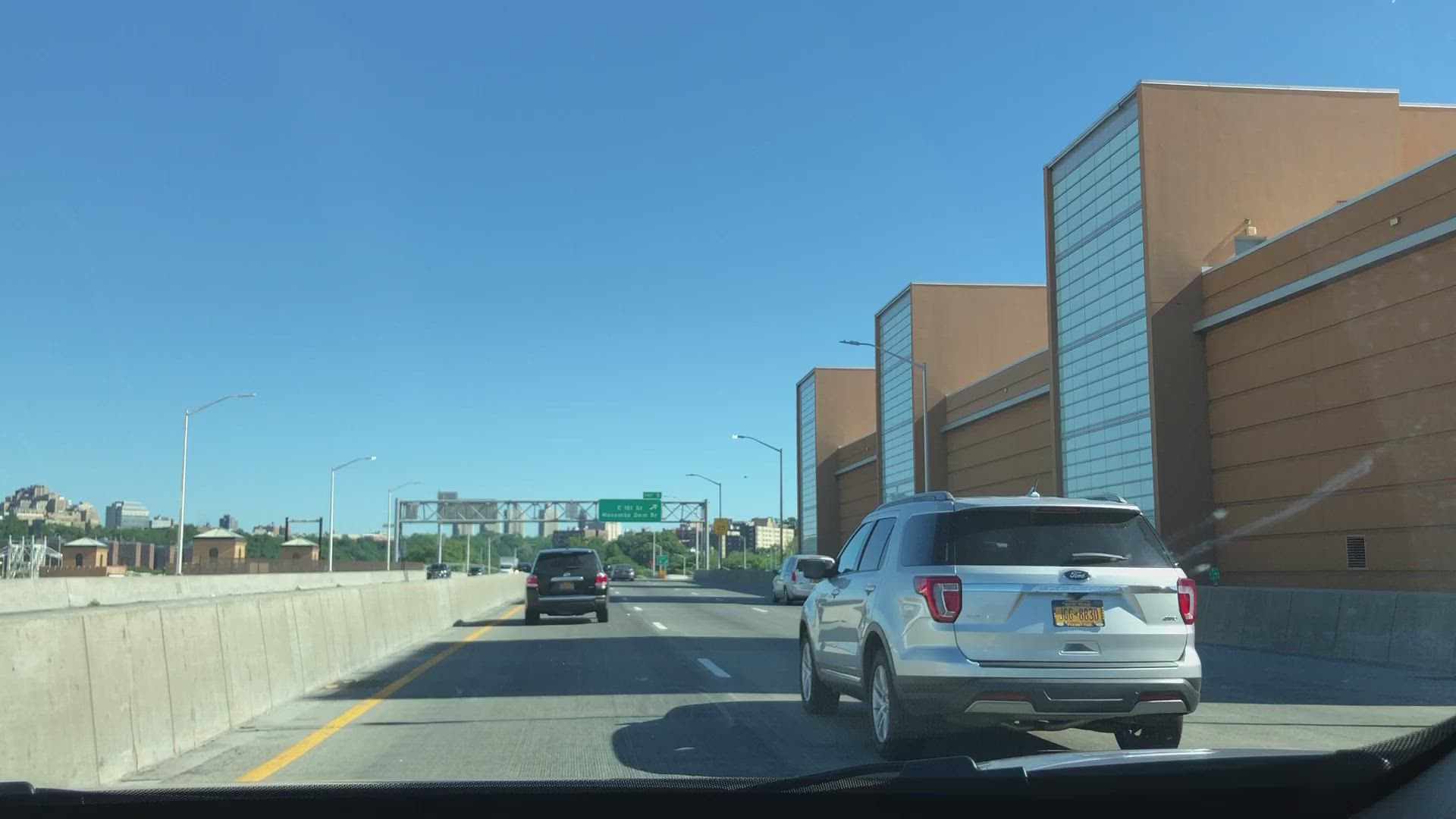A view through the windshield of a moving car shows three vehicles ahead on a three-lane highway. The photo is taken from the perspective of the driver, who is in the left lane. In the middle lane, slightly ahead and to the right, is a darker colored vehicle. Close to this vehicle, there's a silver SUV or hatchback in the right lane. Further ahead in the right lane, a light-colored vehicle is visible. On the right side of the highway, an orange building stands out, while a green highway sign is visible in the distance.